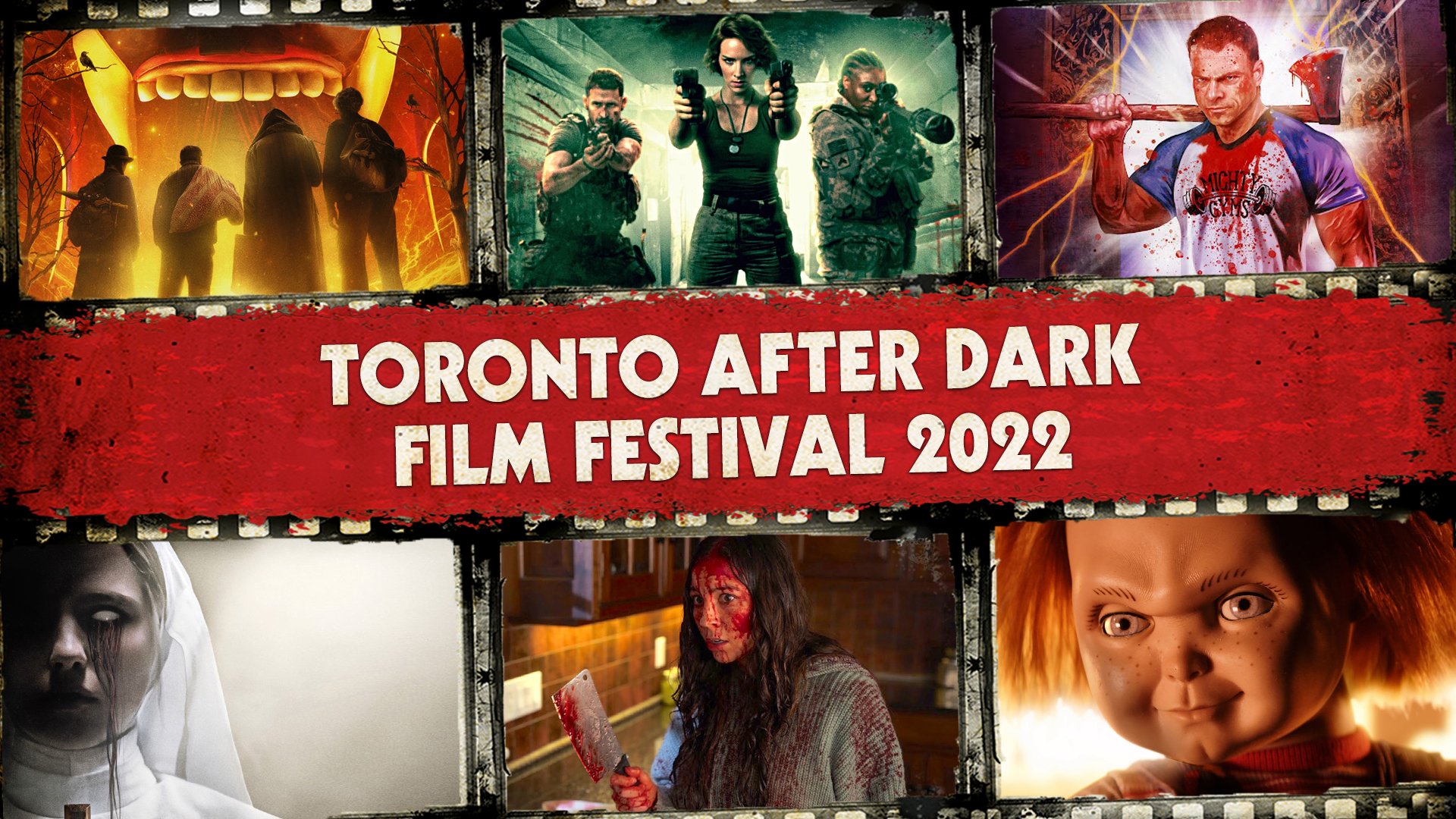This is an advertisement for the Toronto After Dark Film Festival 2022. The central focus of the image is a large, dark red banner with bold white text that reads "Toronto After Dark Film Festival 2022." The banner is framed by what appears to be the edges of a photographic film negative, complete with gaps along the sides. Surrounding the banner are six horror movie screenshots, arranged in two rows of three at the top and bottom of the image. 

Starting from the top left, the first picture shows an ominous scene with an orange background featuring four dark figures entering an open mouth. The top middle picture depicts three military individuals—a man and two women—pointing guns directly at the viewer, with the woman in the middle holding two pistols. The top right image captures a white man in a t-shirt with blue sleeves and a blood-stained chest, holding an axe over his right shoulder.

At the bottom left, there's a haunting image of a nun dressed in a white habit with blood streaming from her left eye. The bottom center showcases a woman with dark hair in a gray sweater, her face and axe both smeared with blood. The bottom right picture features the infamous Chucky doll, glaring menacingly with his signature orangish-red hair and freckled face.